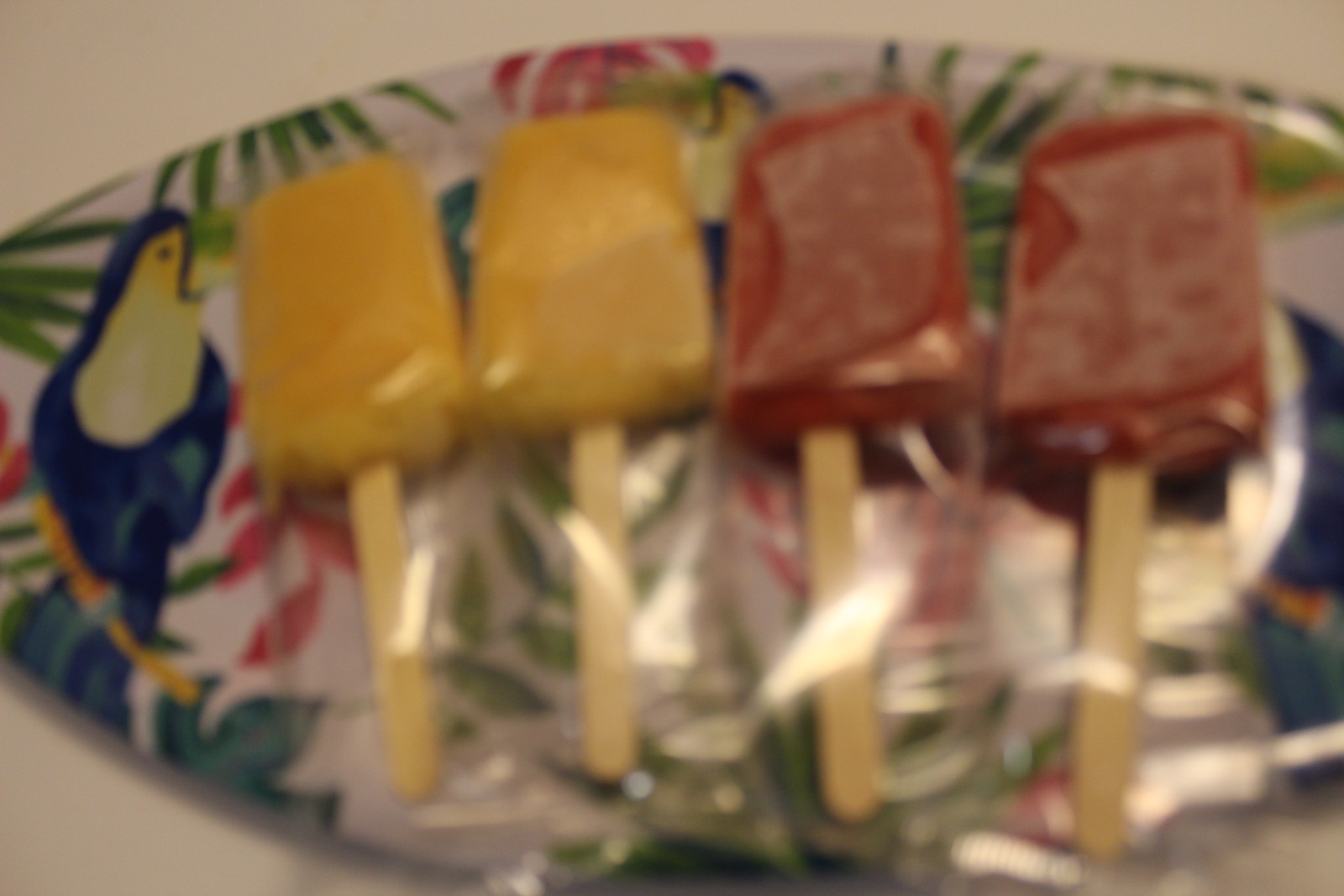This photograph features a slightly blurry image of a long oval plate resting on a beige surface. The plate is decorated with a vivid illustration of blue parrots or parakeets, adorned with yellow and green markings, standing on branches amidst colorful flowers and foliage in shades of red, green, and blue against a white background. Positioned on the plate are four unopened, frost-covered popsicles wrapped in plastic. Two of the popsicles are red, and the other two are yellow, each with a visible wooden stick protruding from the packaging.